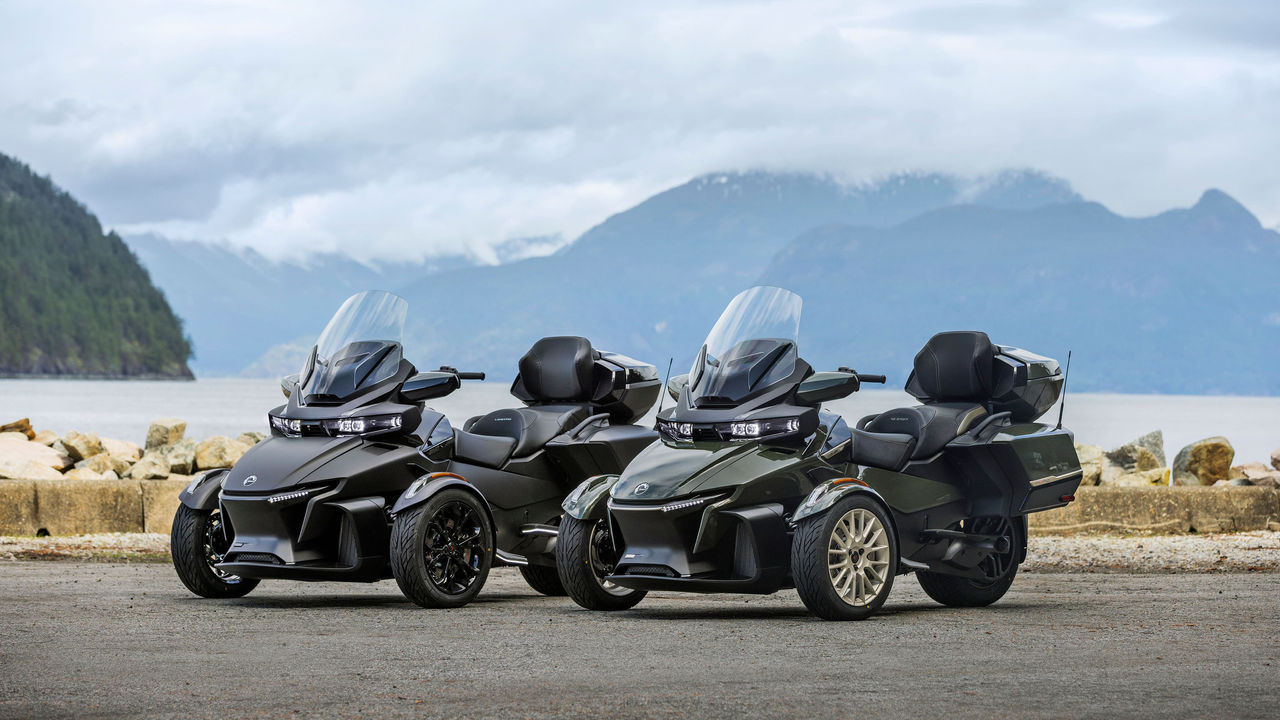The photograph features two three-wheeled motorcycles, often referred to as tricycles or Spyder motorcycles, positioned side by side on a paved roadway. Both vehicles share a two-wheels-in-front, one-wheel-in-the-back configuration. One tricycle is matte black with black rims, while the other is a shiny dark green with golden rims. Both motorcycles are equipped with tall windshields, handlebars, and large storage compartments or saddlebags at the rear. The background reveals a scenic outdoor setting, with a rocky divider separating the roadway from a body of water. Towering above the water are majestic mountain peaks, partially obscured by low-hanging clouds. To the far left, one of the mountains is lush with dense greenery and trees. The sky overhead is filled with white, puffy clouds, adding to the picturesque landscape. The overall ambiance suggests a locale of considerable natural beauty, possibly the Rocky Mountains, creating a promotional feel to the image.